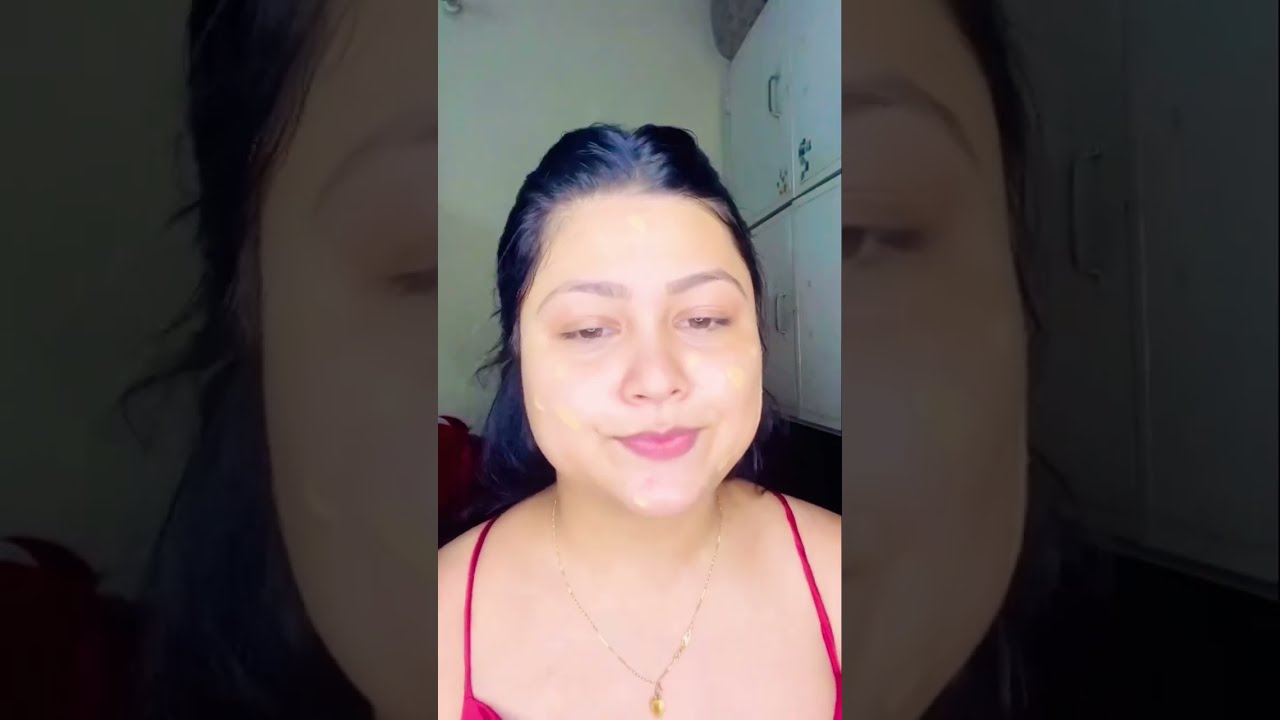The image appears to be a screen grab from a vertical TikTok-style video featuring a young woman in her mid-twenties. She has a round face with dark black hair pulled back, possibly into a ponytail or bun, and is wearing pink lipstick. The lighting gives her hair a slight purple tint. She’s dressed in a red spaghetti strap tank top and adorned with a gold necklace with a pendant. The woman, who might be Asian, has a neutral expression, as if she's mid-sentence, and her brown eyes are partially closed, looking slightly off-camera. The background suggests she's in a bedroom, with white or off-white walls, white cabinets, and some possibly written-on white surfaces. The image is presented in a triptych format, where the center panel shows the full image while the left and right panels are zoomed-in sections of the left and right parts of the center image, respectively.